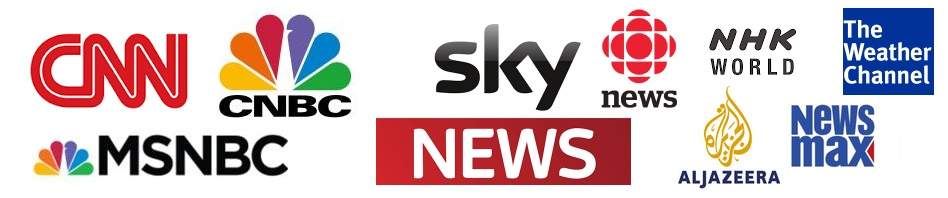The image features a clean, white background showcasing a collection of nine distinctive news outlet logos. The prominent logos include CNN in its signature red, CNBC represented with its colorful peacock emblem, Sky and Sky News, each sporting a modern design. Also present is NHK World, The Weather Channel in its recognizable blue, Newsmax, Al Jazeera with its elegant Arabic script, and MSNBC. Each logo is clearly displayed, offering a visual index of these well-known news organizations. The stark white backdrop keeps the focus solely on the logos, allowing viewers to easily identify each brand. The collection is comprehensive, featuring major global and U.S.-based news sources, although one logo simply labeled "News" appears generic and less identifiable. This array highlights the visual trademarks of these staple news outlets.